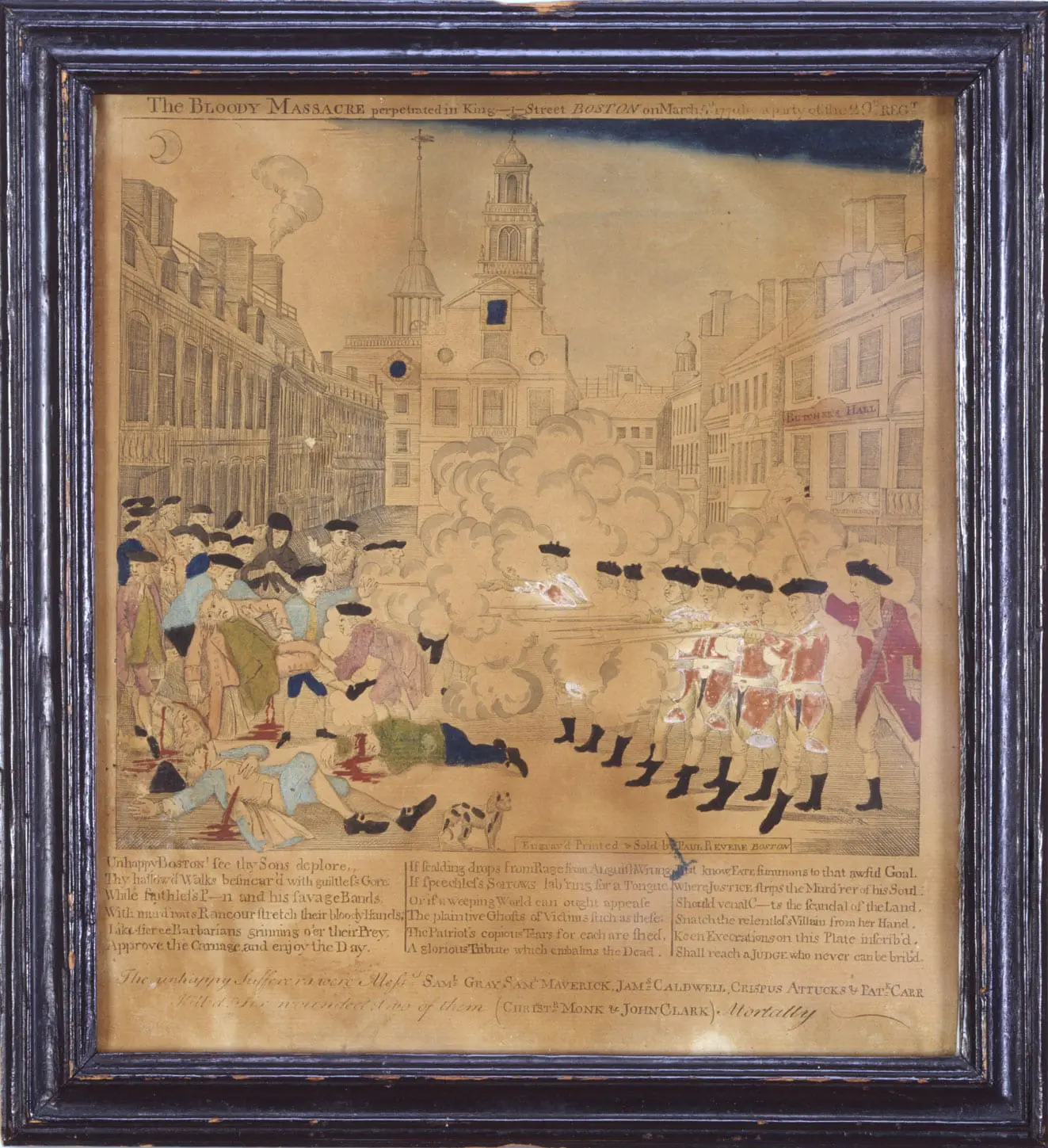This framed image, titled "The Bloody Massacre," is a weathered historical print likely depicting a scene from the Revolutionary War. The frame itself is an old, beveled wood, painted black with chipped areas, giving it a distinctly antique appearance. The browning and wrinkled paper inside the frame, looking like an aged newspaper, reveals a hand-drawn illustration of British soldiers in their iconic red coats firing their muskets. The chaotic battle scene unfolds with billows of smoke at the center, and anguished figures in regular street clothes on the left, visibly wounded and bleeding profusely. The grim scene is set against a backdrop of period buildings lining a street, emphasizing the urban nature of the conflict. Below the depiction, the title is prominent: "The Bloody Massacre," with additional text that includes the date, "perpetrated in King Street, Boston on March 5th," and a partial credit to John Clark among other unreadable inscriptions.